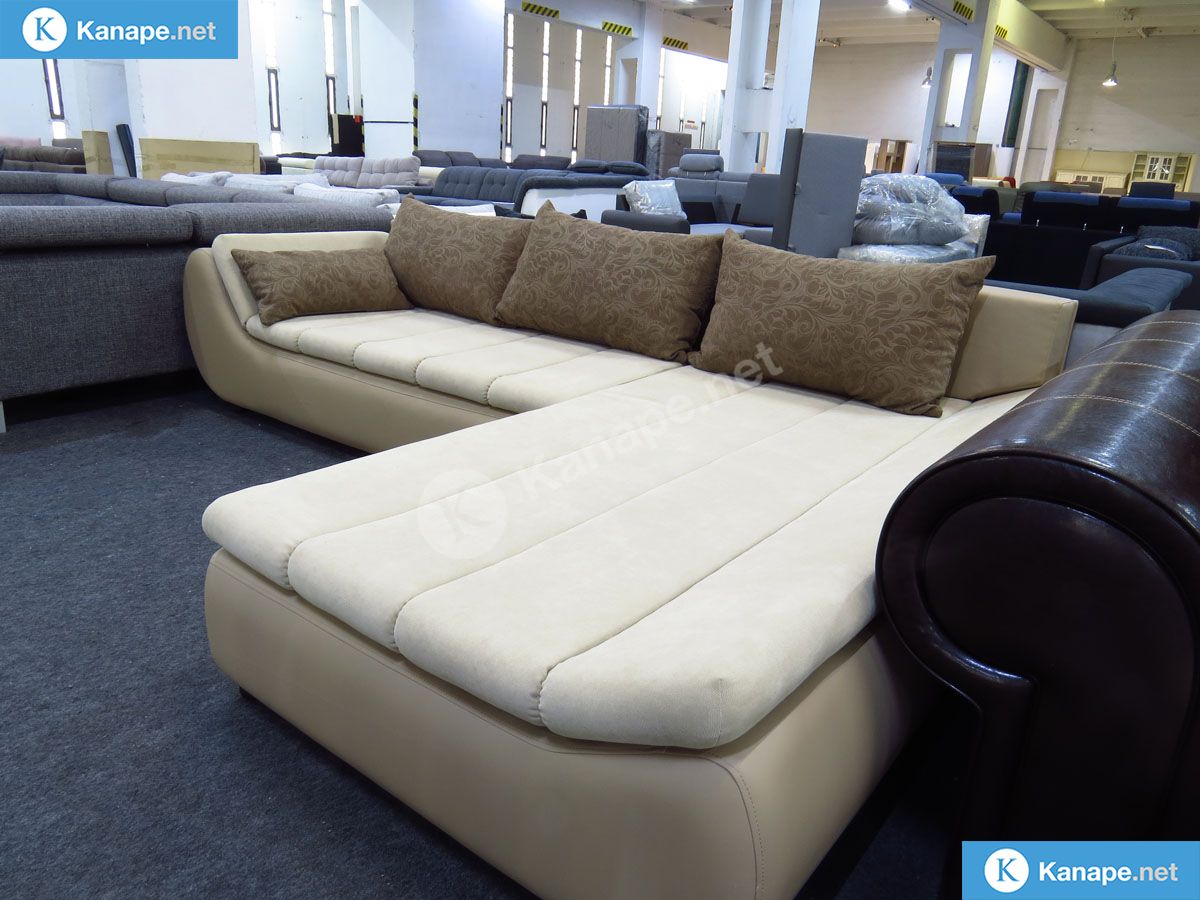The photograph depicts a bustling furniture showroom filled with an assortment of couches. The focal point is a distinctive, L-shaped sectional sofa framed in a beige/tan leather-like material, resembling an airbed on the bottom layer. The top part of the sectional is upholstered in an off-white fabric, giving it a unique two-piece look. The surface is gently scooped rather than featuring traditional armrests, adding an intriguing design element. This sectional is adorned with three large brown fabric pillows along the backrest and an additional smaller rectangular brown pillow placed at the left side or arm of the couch. In the background, the expansive showroom is filled with various other couches, including a glimpse of a rolled arm sofa with a windowpane plaid pattern. At the top left and bottom right corners of the image, a logo featuring a blue rectangle with a blue 'K' inside a white circle can be seen, accompanied by the text "K-A-N-A-P-E dot net."